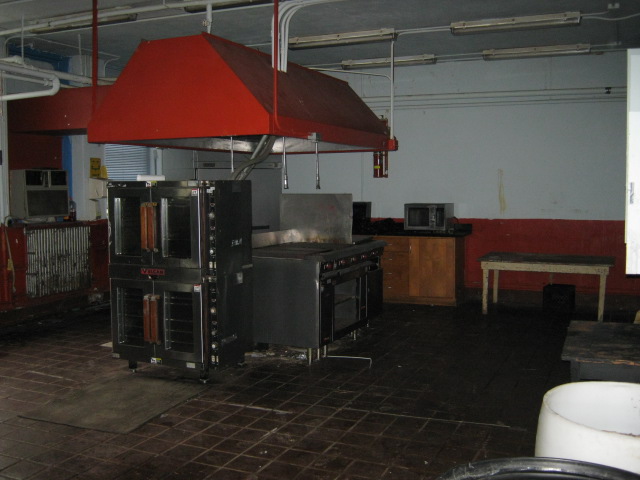The image depicts the interior of an old and likely out-of-use restaurant kitchen. Dominating the center of the room is a large, red ventilation hood hanging from the ceiling, situated above professional-grade stoves with wide burners. Adjacent to the stoves are stacked ovens or heating containers, adding to the industrial ambiance. The kitchen's equipment is primarily black and gray, with additional metal heating racks or storage units featuring round handles. The decor includes gray walls with red trim and brown cabinets, contributing to the overall aged and grimy appearance. The floor, stained with dirt and grime, features a dark brown towel and a black rug. The space is dimly lit, emphasizing the neglected state of the kitchen.